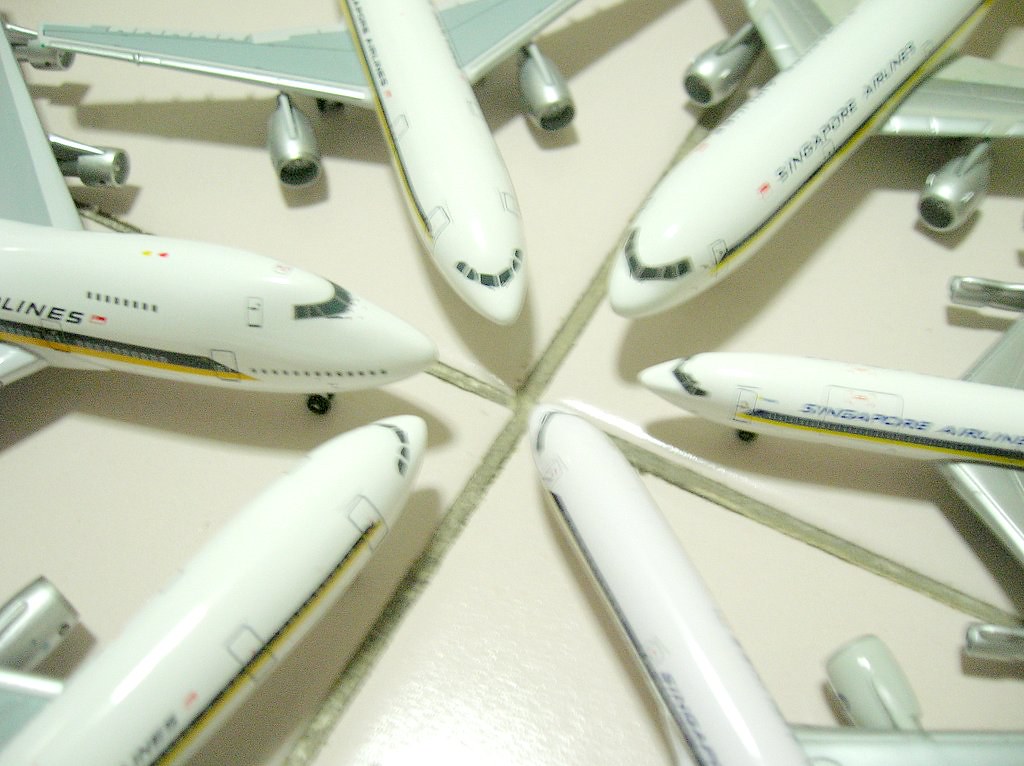The photograph is an indoor color image showcasing six highly detailed model planes arranged in a circular pattern on a tiled floor. The planes, painted in the distinctive white livery of Singapore Airlines with varying pinstriping in blue, yellow, and black, and bearing the airline's name on their sides, are modern jumbo jet styles, including models like the Boeing 747, Boeing 777, and Airbus. The planes' noses point inward towards the center of the image, where the corners of four large, off-white ceramic tiles meet, forming a cross of mid-grey grout. The scene is slightly out of focus, suggesting it was taken with a cell phone or similar device, and the cropping of the image allows only the front halves of the planes and glimpses of their silver-tone wings and engines to be visible. The overall composition and details suggest a display of collector's model planes.